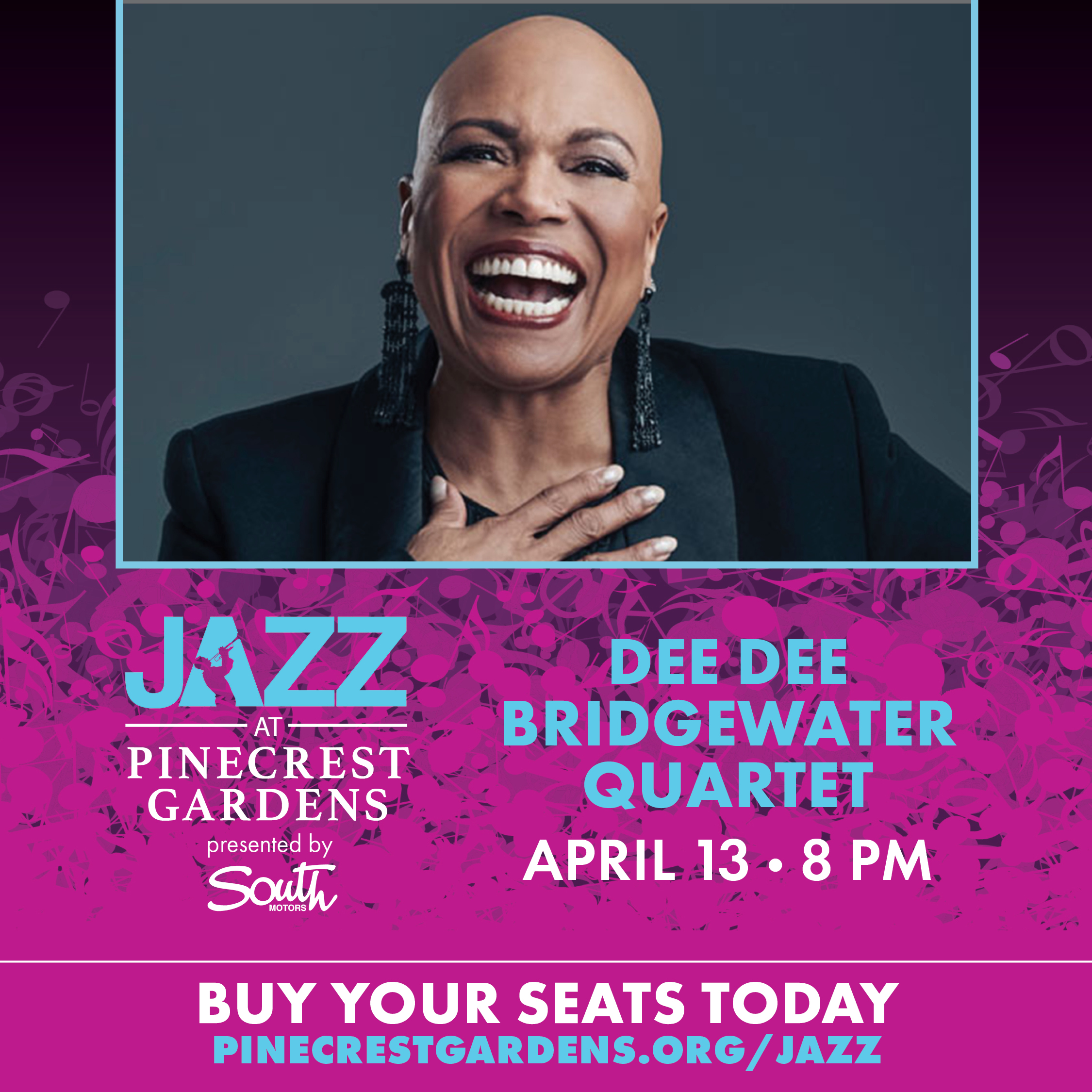This vibrant, modern poster advertises the Dee Dee Bridgewater Quartet's upcoming jazz concert at Pinecrest Gardens, presented by South Motors. The image features a striking, bald African American woman, Dee Dee Bridgewater, dressed in an elegant black tuxedo jacket with satin lapels. She exudes charisma with her wide, joyful smile, accented by bold red lipstick and long, drop earrings that nearly touch her shoulders. Her left hand is placed over her chest, enhancing the warmth of her laugh. The background of the image where her portrait is placed is a contrasting dark teal-green, while the rest of the poster is a lively purple-mauve. The text is a mix of blue and white fonts and includes key details: "Jazz at Pinecrest Gardens," "Dee Dee Bridgewater Quartet," the concert date "April 13th at 8pm," and a call to action, "Buy your seats today" with the ticket link "pinecrestgardens.org/jazz." The overall design blends modernity with a captivating aesthetic, reflecting the energy and sophistication of the jazz event it promotes.